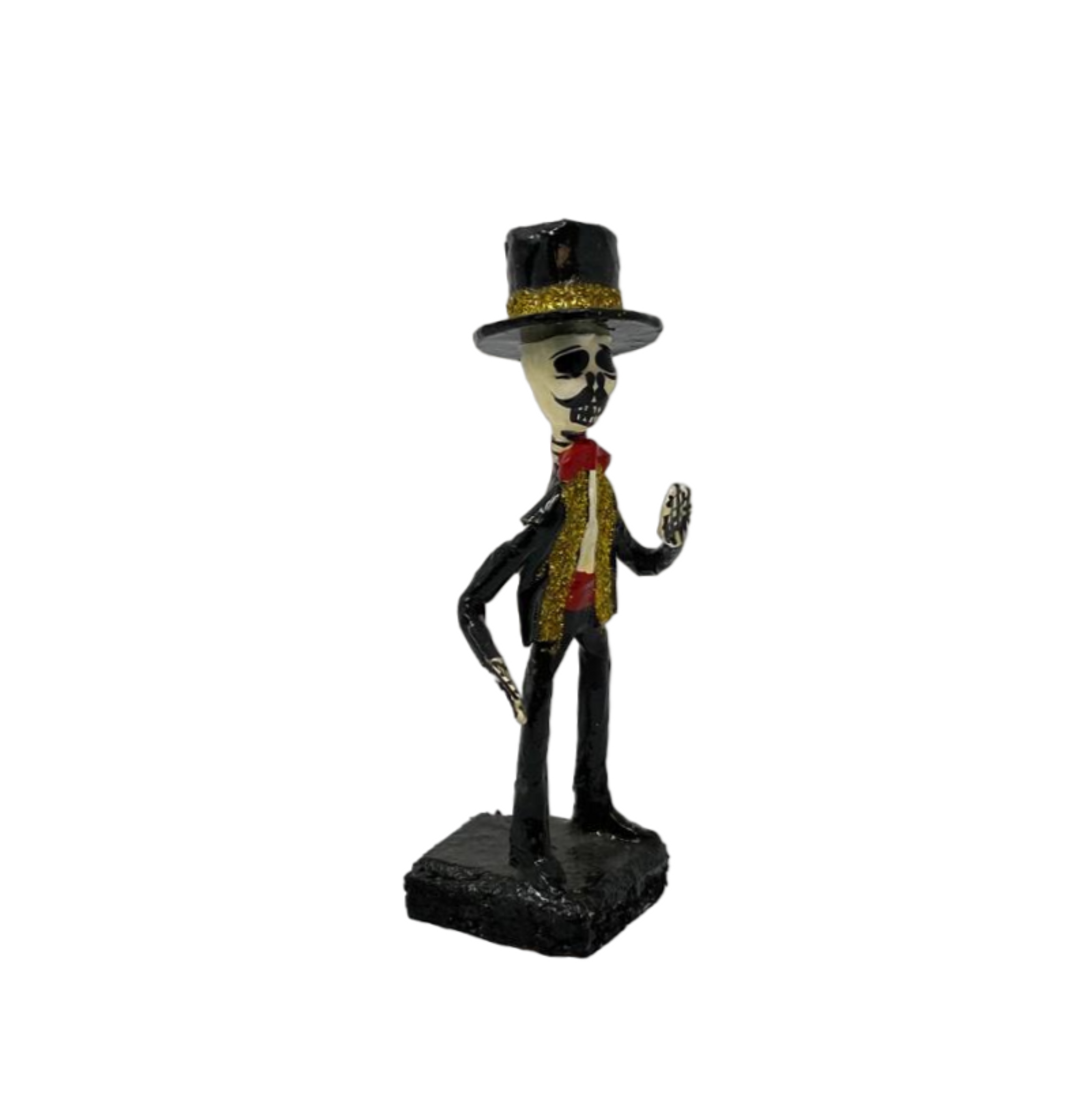This image depicts a detailed figurine, likely commemorating the Mexican Day of the Dead celebration. The small statue stands on a shiny black platform with a tar-like sheen. Crafted from metal and possibly clay, the skeletal figure is dressed in an elegant bullfighter's attire. It dons a black jacket with gold glitter lapels, a white shirt, a red bow tie, and a matching red cummerbund. Its clothing ensemble is completed with black pants. The skeleton features stark black detailing on its white hands, resembling skeletal bones. The figure's face, a skeletal white with solid black eye sockets, distinct teeth, and a black mustache, adds to its festive appearance. It wears a black top hat adorned with a gold glitter band. The left hand is raised in a wave, while the right hand rests casually against its right leg, making it a captivating and culturally rich representation.